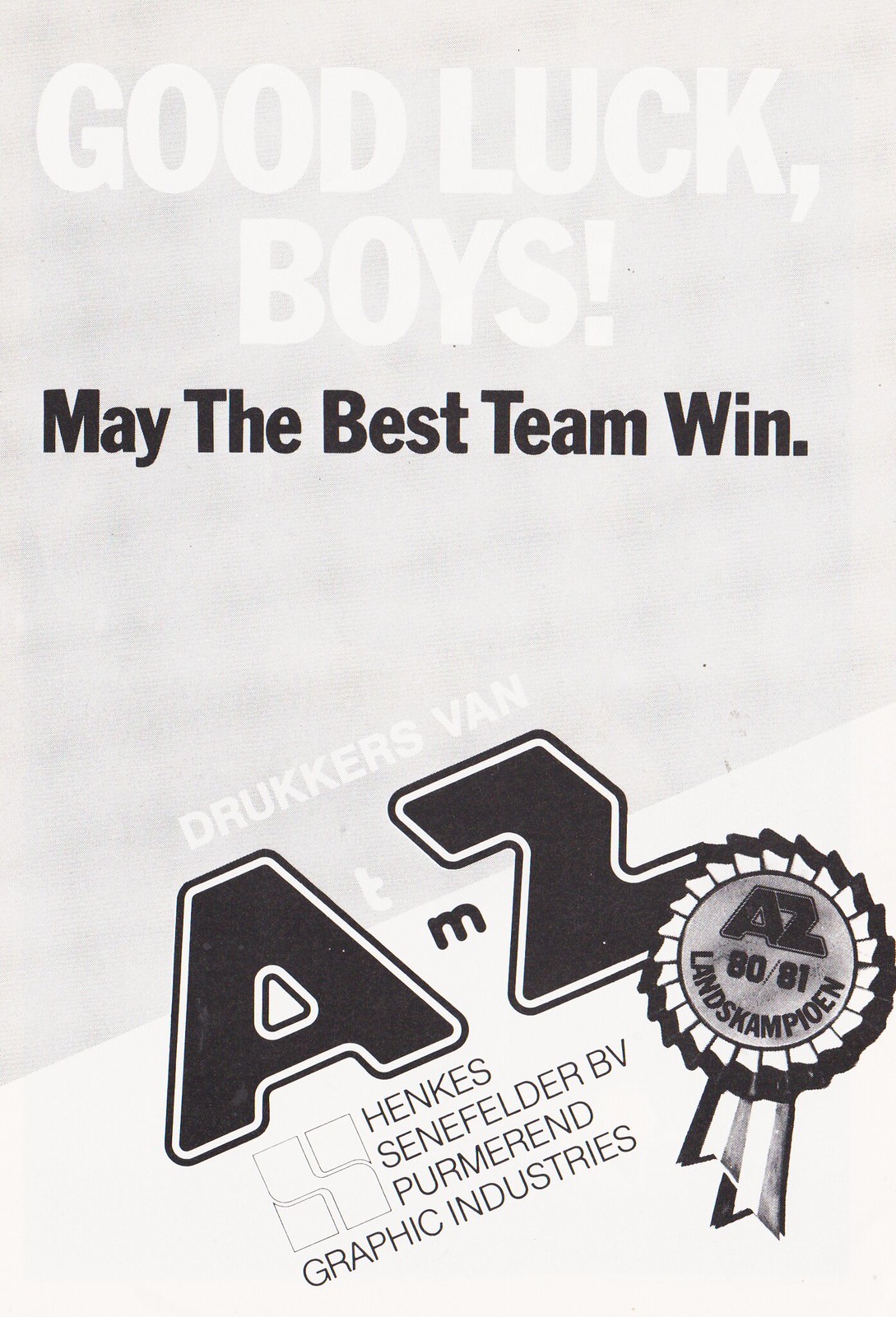This black-and-white image depicts a morale-boosting sign or banner for a sports team. The background is largely a light gray, with white text at the top that reads "Good luck boys," followed by "May the best team win" in black text. Toward the bottom, in white text that nearly blends into the gray background, is "Drucker's Van." Dominating the middle section in large, bubbled black letters filled with white ink are the initials "A" and "Z." Below the "A," four checkboxes are visible next to the words "Henke's Sennfelder BB, Permanent Graphic Industries." Adjacent to the "Z" is a prominent black-and-white ribbon inscribed with "AZ-8081, Landskampion," likely referencing a championship. The overall image is devoid of people and features a predominantly gray backdrop.